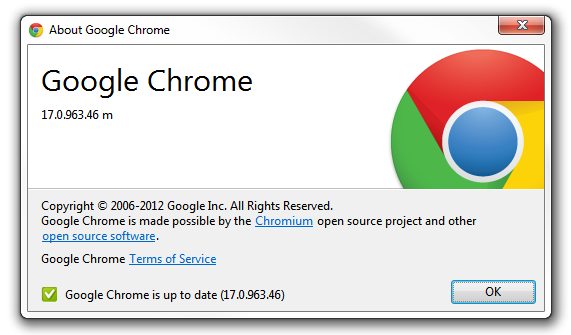The image depicts an old version of a Windows pop-up notification box, characterized by a shadowed border and a close icon in the upper right-hand corner, identifiable by a small red button. At the top of the box, it is labeled "About Google Chrome" alongside the Chrome icon. The version number "Google Chrome 17.0.963.46" is prominently displayed.

In the right section of the pop-up, there is a partially visible, enlarged Google Chrome icon. The icon's red, green, yellow, and blue segments are visible, though the bottom and far right portions are cut off. Beneath this visual, a darker gray bar features black textual elements stating, "Copyright 2006-2012 Google Inc. All rights reserved."

Further details within the text mention that "Google Chrome is made possible by Chromium," with "Chromium" styled in blue, underlined text, signaling a clickable link. Additionally, it references the "Open Source Project and other open source software," where "open source software" is similarly styled in blue and underlined. Another clickable link, "Google Chrome Terms of Service," is also underlined in blue.

Below these descriptions, a small green checkmark box asserts, "Google Chrome is up to date (17.0.963.46)." On the right-hand side, an "OK" button bordered by a blue edge and featuring black text provides an action option. The entire pop-up box is outlined by a thin gray line that extends from the top, just under the "Google Chrome" text, to the bottom, including a division beneath the enlarged Chrome icon.